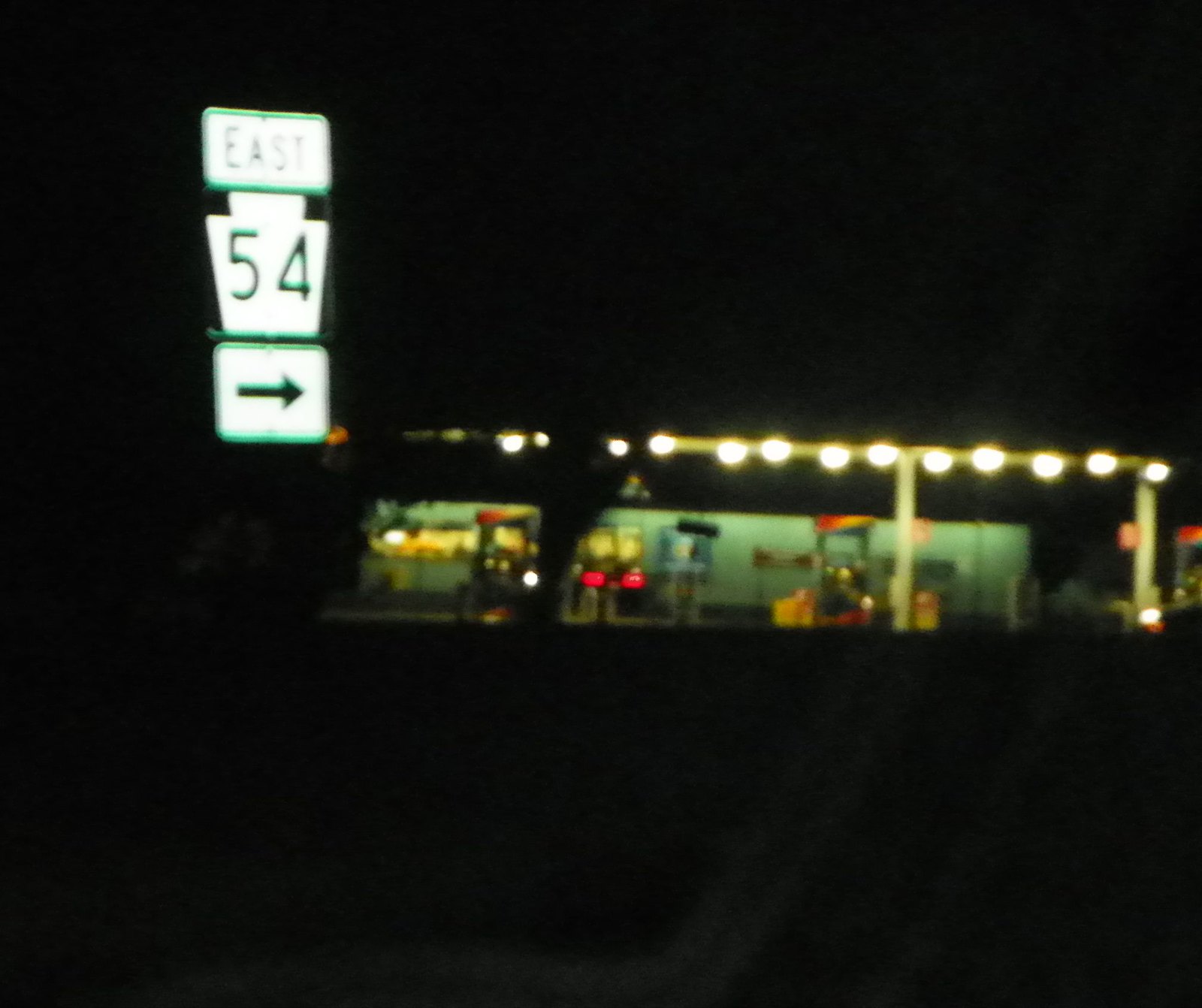The image depicts a nighttime scene at a gas station, captured with a low-quality camera resulting in significant motion blur and a lack of focus. To the left of the frame, a sign marked "East 54" with an arrow pointing right is partially visible. The gas station building, possibly mint green in color though it might be a trick of the lighting, features several illuminated gas pumps. Bright white lights line the roof of the gas station, standing out starkly against the darker background. A few cars are present, identifiable only by their red taillights and white headlights piercing through the blur. The overall lighting creates a somewhat surreal and hazy atmosphere, accentuated by the motion blur across the scene.